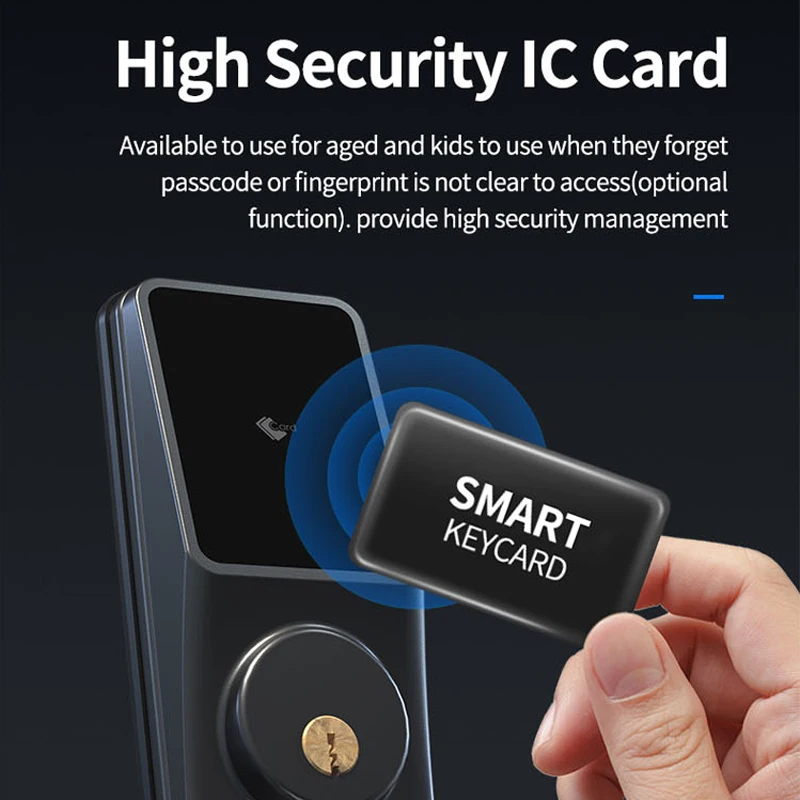The image features a High Security IC Card system, prominently displayed against a gray background. At the top, large white letters read "High Security IC Card." Beneath this, smaller white text details that the card is "Available to Use for Aged and Kids to Use When They Forget Passcode or Fingerprint, Is Not Clear to Access, Optional Function, Provide High Security Management." On the left side, a rectangular smart lock panel is shown, which includes an area to insert the smart card or a numerical keypad. Towards the bottom of the panel is a keyhole, designed as a backup access option. An accompanying graphic shows a blue circle radar effect emanating from the card. On the right side of the image, a hand is holding up a black and gray Smart Key Card with white writing, positioned as if it is about to interact with the smart lock panel.